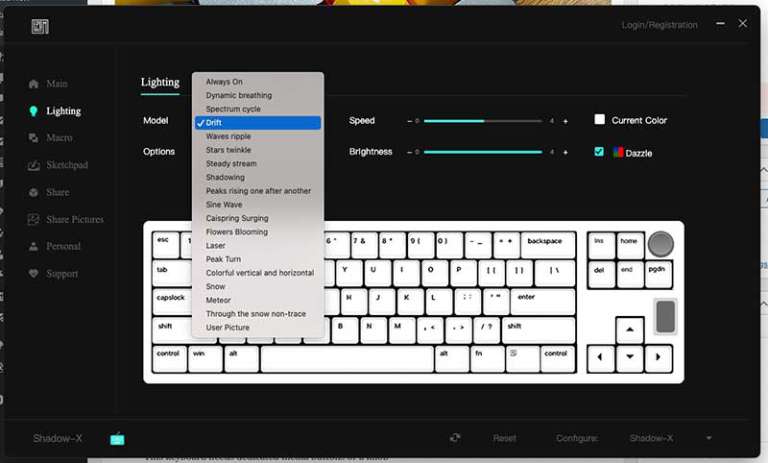This image appears to be a cluttered screenshot from a website or a software user interface, showcasing multiple overlapping windows featuring various controls and settings. The background of the primary window is black, adorned with white text. However, the clarity is compromised due to the image's resolution, requiring zooming to decipher the details. 

At the top of the image, a horizontal band with grey, yellow, and white colors is present, serving as a background. On the right side of this band, a portion of a graph with a blue header is visible, albeit partially obscured by another window.

On the right-hand side of the main window, there are greyed-out options for "login" and "registration," indicating user authentication features. The window's black background hosts a vertical list of text alongside icons on the left side. Among these, the "Lighting" section is especially highlighted in green. The other legible sections include "Music," "Macro," and "Shuttle Pad," although many are too poorly rendered to read.

The open "Lighting" tab reveals various settings such as "models," "options," "speed," "brightness," and additional controls like "current color" and "dazzle." Within this main window, two smaller, overlapping windows are evident. 

One of these additional windows appears to be a keyboard interface, possibly an on-screen keyboard, characterized by white keys outlined in black. The second overlay resembles a context menu typically seen when right-clicking, featuring options like "Always on," "Dynamic breathing," "Spectrum," "Cycle," and other lighting effects such as "Drift," which is highlighted in blue, "Wave," "Ripple," "Stars," and "Twinkle," among others.

This intricate layout of multiple windows and settings tabs creates a complex and crowded visual depiction, highlighting the extensive customization and functionality being showcased.